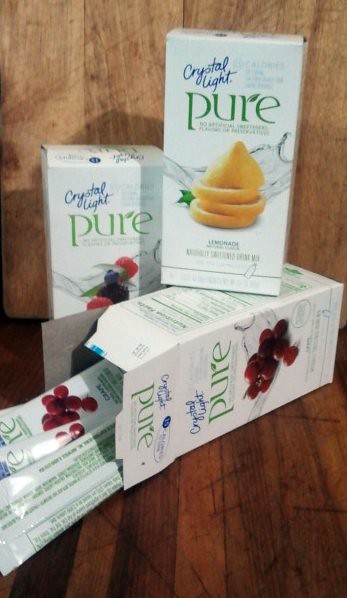This photograph features a trio of Crystal Light Pure boxes arranged on a wooden surface. The background wood is a lighter, warmer tone, while the wood below is a deeper, richer shade. Each small, white cardboard box, estimated to be about three and a half inches tall by two inches wide, contains water flavoring additives.

The box on the bottom, which appears to be a cherry flavor, has been opened, spilling its contents towards the front left of the image. Above it, positioned diagonally, is the lemonade-flavored box, identified by the bright yellow color and an illustration of chopped lemons. The third box, likely mixed berry flavor with raspberries depicted on it, stands behind the other two, partially obscured.

All three boxes share a consistent design: the words "Crystal Light" in blue lettering, and "Pure" in green, highlighted by a note indicating the products contain no artificial sweeteners. The vivid imagery and varied positioning of the boxes convey a sense of casual disarray, making the scene appear both dynamic and visually engaging.